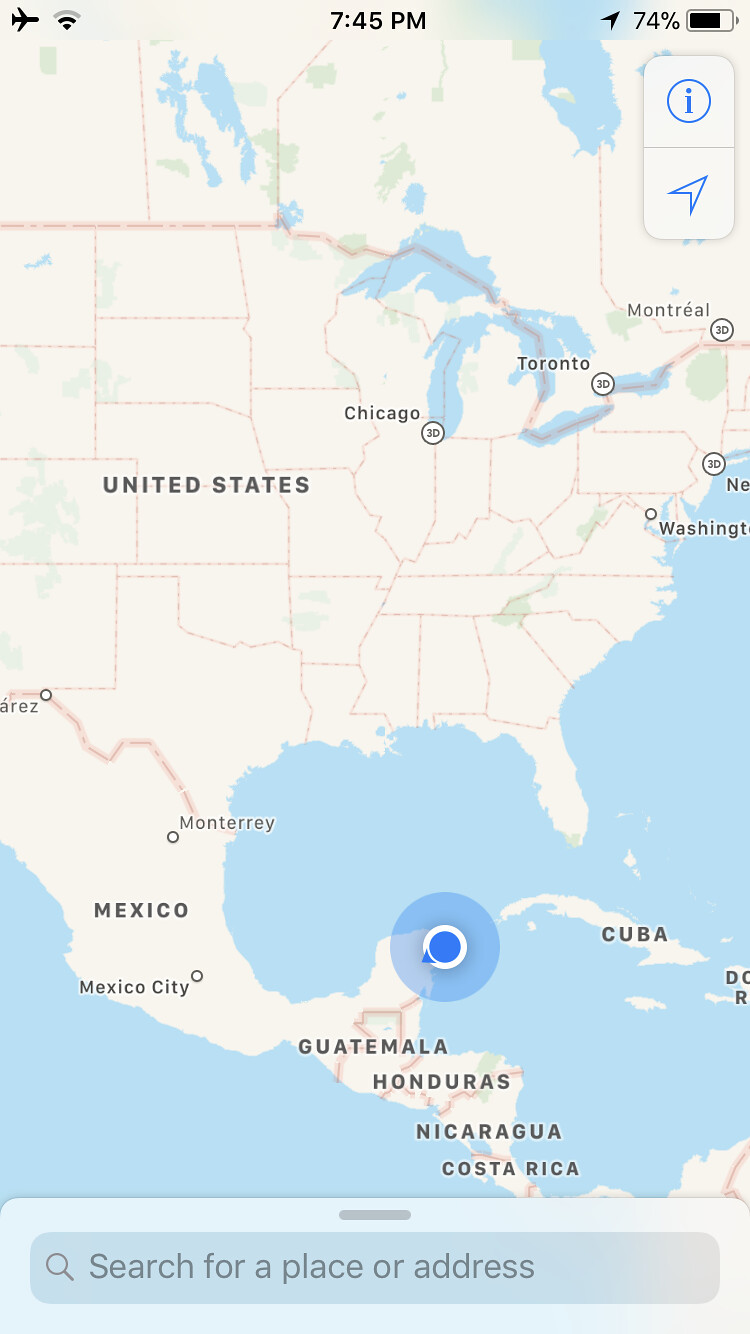Screenshot of a smartphone displaying the Google Maps interface. At the very top of the screen, there is an airplane mode icon on the left, followed by a Wi-Fi or signal strength icon. On the right, a battery icon indicates the remaining battery life. The time, 7:45 PM, is displayed in the center of the status bar. The main content of the screen shows a map of North America with a map pin marking a specific location in southern Mexico.